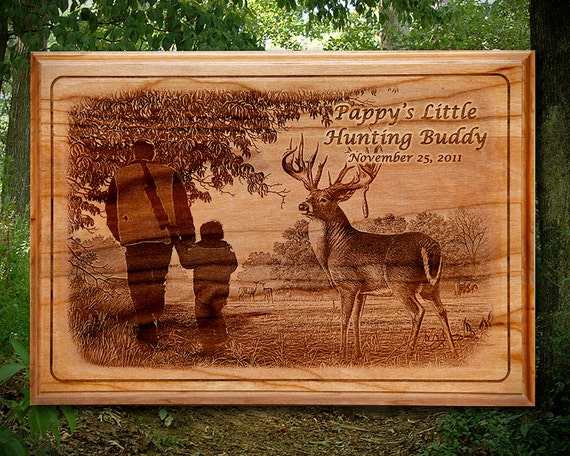The image depicts a large, laser-engraved wooden cutting board, presumably a present, placed against a natural outdoor backdrop featuring a woodsy scene with trees, greenery, and a dirt path. Central to the cutting board is an intricate engraving showing a grandfather and his grandson, viewed from behind as they walk hand-in-hand from a field into a forest. The older man carries a hunting rifle slung over his shoulder, suggesting they are on a hunting trip. Dominating the scene next to them, albeit in an unrealistic proximity, is a prominently featured male deer with an impressive set of antlers. The cutting board is inscribed with the text "Pappy's Little Hunting Buddy, November 25, 2011," enhancing its sentimental value. The detailed engraving also includes surrounding elements like trees and grass, creating a cohesive, heartwarming depiction of a bonding moment set in nature, possibly meant to celebrate or memorialize a special occasion or tradition related to hunting and family.